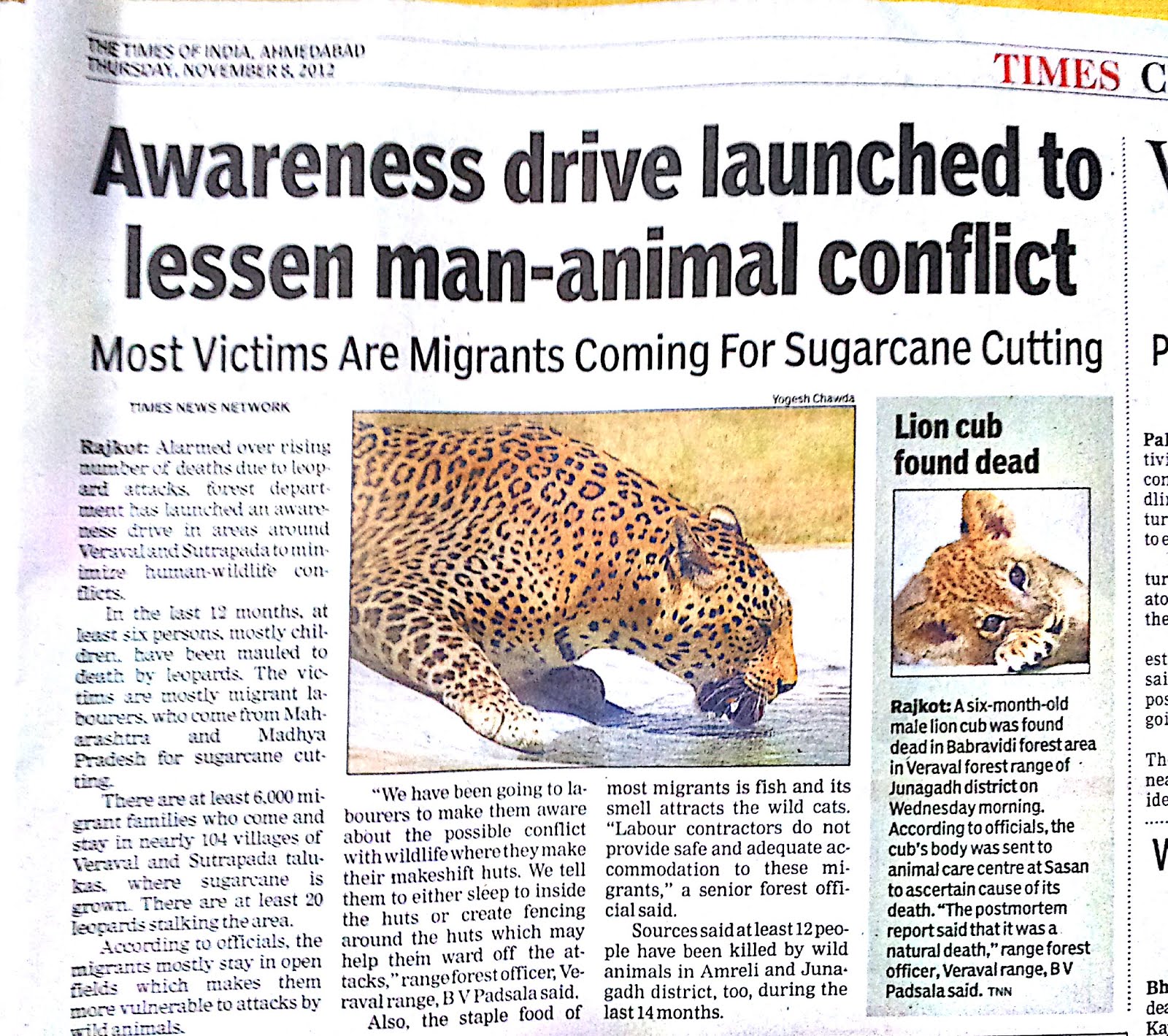The image appears to be a scanned or uploaded newspaper page from *The Times of India*, specifically the Ahmedabad edition, dated Thursday, November 8, 2012. The main headline, prominently displayed, reads: "Awareness Drive Launched to Lessen Man-Animal Conflict."

Underneath, a subheadline addresses the issue: "Most Victims are Migrants Coming for Sugarcane Cutting," highlighting the demographic most affected by the conflict. The accompanying photograph shows a leopard drinking water, symbolizing the wildlife involved in these incidents. The caption beside the image notes: "Raghjot – Alarmed Over Rising Number of Deaths to Leopards and Attacks, Forest Department Has Launched an Awareness Drive in Areas Around Vrishapudra Where Human-Wildlife Conflicts."

Although the text appears slightly blurry, likely due to scanning issues, another article on the same page reports on a tragic wildlife discovery. The headline reads: "Lion Cub Found Dead in the Same Area." The article details the finding of a six-month-old male lion cub in the Bravarti Forest Area and Vrishapudra Forest Range of the Jhangashtriya on Wednesday morning. Officials sent the cub’s body to the Animal Care Center at Sasan for a post-mortem, which concluded that the cub died a natural death, as stated by Range Forest Officer, B.V. Pisada.

The image also reveals another partially visible page of the newspaper, characterized by dotted lines, though much of its content is obscured or cut off.